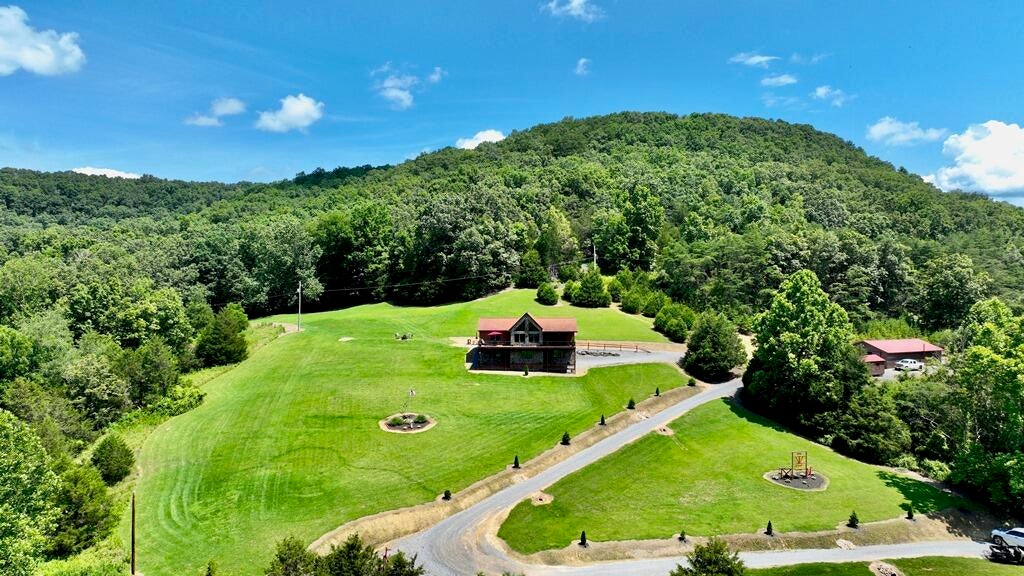A bright and vibrant aerial photo showcases a serene, rural landscape taken during what appears to be the afternoon on a sunny day. The upper fourth of the image is dominated by a clear, blue sky dotted with a few small, white clouds. Below, the hills are densely covered with lush, green foliage, almost resembling a thick forest. In the center of the photo lies a large, flat, meticulously mowed grassy clearing. 

At the heart of this clearing stands a grand, two-story, Victorian-style house with a distinctive gabled, red roof. The house itself features a brown exterior and is accentuated by its large presence in the serene setting. A winding road leads to the house, bordered by small, newly planted trees. 

To the right of the central house, partially obscured by the surrounding trees and bushes, there is another smaller red structure, possibly a guest house or a shed, with a pickup truck parked nearby. Additionally, towards the bottom right of the image, near where the road curves, a white truck can be seen. The entire scene exudes peace and tranquility, framed by the vivid greens of the grass and trees and the deep blue of the sky.